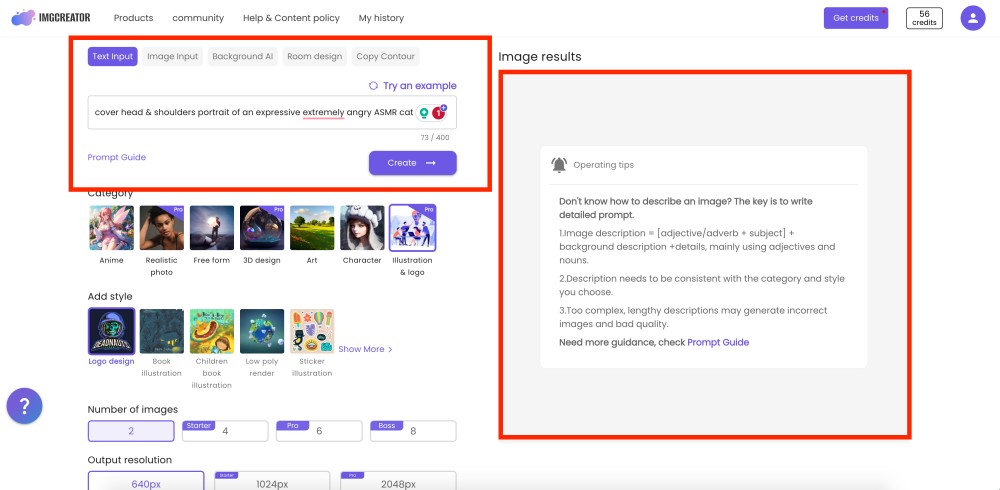This image showcases the interface of the IMGCREATOR website.

In the upper left-hand corner, the website's name, "IMGCREATOR," is prominently displayed. Adjacent to this, there is a menu presented in a gray font, featuring the following options: Products, Community, Helping, Content, Policy, and My History. Below this menu, a highlighted red box contains multiple buttons arranged vertically. The buttons are labeled as follows: Text Import, Image Input, Background AI, Room Design, and Copy Contour. Beneath these buttons, there's a clickable option labeled "Try an Example."

In the center of the interface, there is a prominent search bar. This bar displays an example input: "Cover Head and Shoulders Portrait of an Expressive Extremely Angry ASMR Cat." Next to this search bar is a large "Create" button, encouraging user interaction. Below this, the Category section can be found, showcasing a list of categorized examples such as Anime, 3D Design, Art, and Character.

This detailed everything provides a clear understanding of the navigation and tools available within the IMGCREATOR website interface.